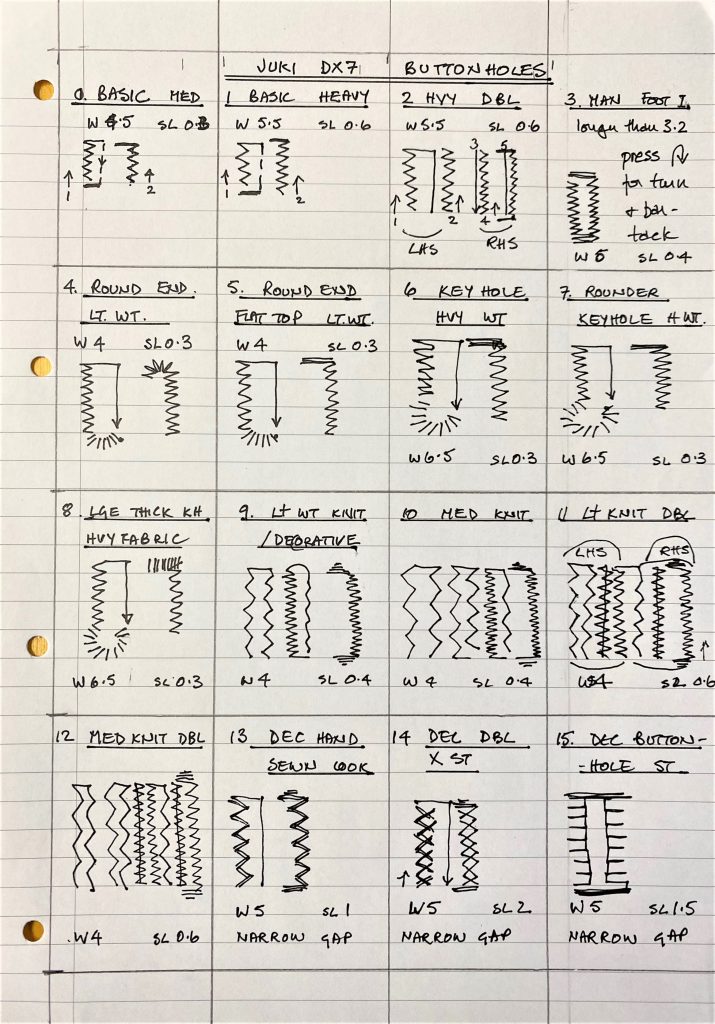The image captures a color photograph in portrait orientation, featuring a piece of lined notebook paper with black handwritten ink notations. The paper is standard with three hole punches along the left margin, displaying a beige background through the holes. The sheet is meticulously divided into a table with 16 boxes, arranged in four columns and four rows. Each box contains technical illustrations and text, marked with numbers starting from 0 in the top left corner, progressing horizontally and ending with the number 15 in the bottom right box.

At the top center of the page, a headline is double-underlined, prominently displaying "JUKI DX7 button holes!" The divisions appear to be homemade, with hand-drawn lines creating the grid. The notations within each box include labels and crude drawings resembling electronic circuits with jagged and straight lines. Some discernible text in the boxes includes "basic med" in the first box, "one basic heavy" in the second, and "two H-V-Y-D-B-L" in the third. The detailed drawings and text in each box reveal a mix of technical specifications and design notes, interspersed with zigzag lines and additional marginal texts.